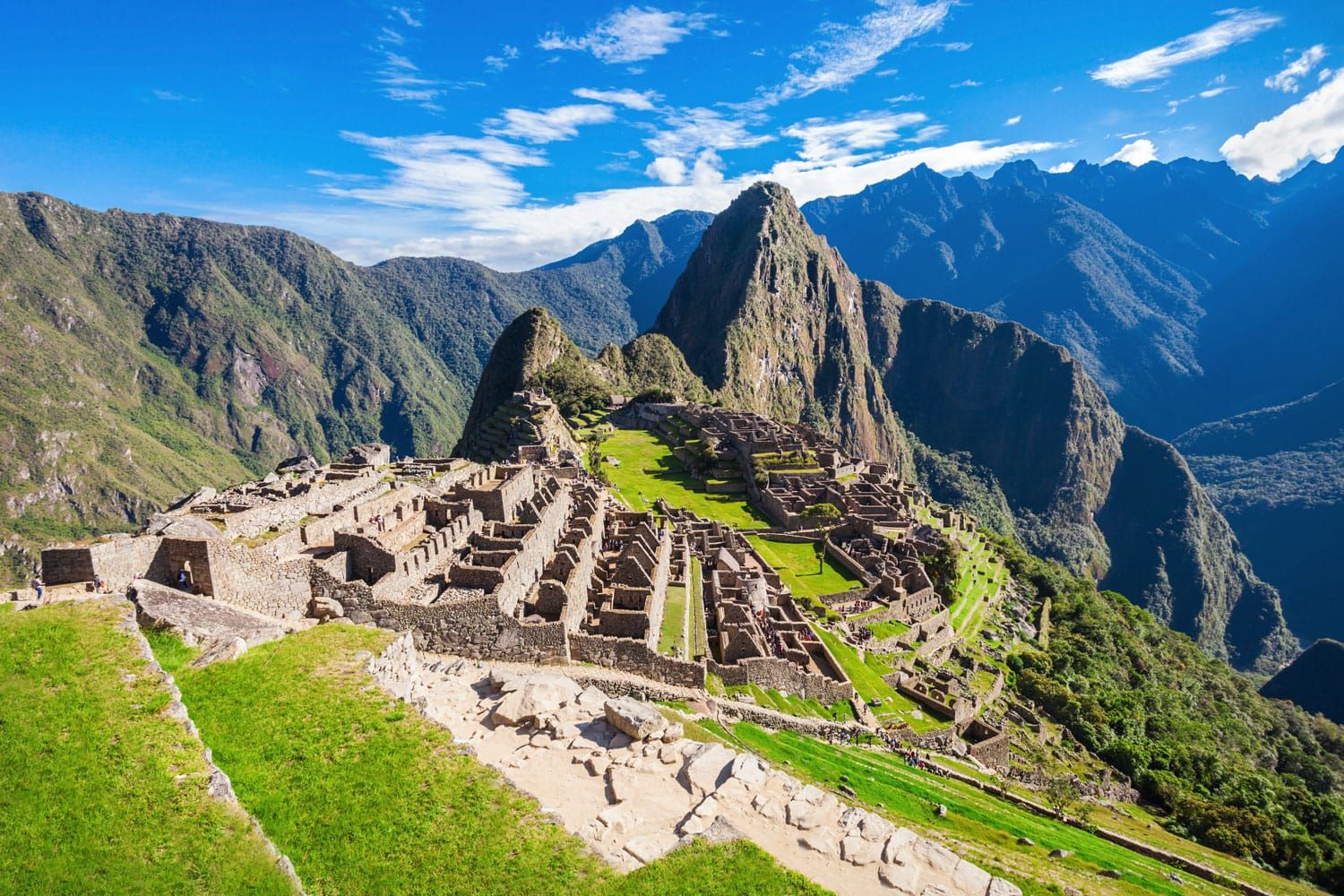The image depicts a breathtaking landscape, featuring an ancient archaeological site reminiscent of Machu Picchu. In the foreground, there is a hill overlooking a series of historical ruins. These ruins consist of multiple buildings constructed from white and brown bricks, arranged in four to five staggered rows without roofs. Descending the hill, one can see grassy steps and stone pathways leading towards the bottom right. In the center of the image lies an amphitheater-like area with verdant green grass and stone seating that ascends about five or six levels.

To the left, additional ruins and grassy terraces appear, adding layers to the scene. The middle section reveals remnants of a village, similarly made of connected buildings in ruins. As the eye moves towards the background, the towering mountains become more prominent. A mountain wall arcs over the village, creating a dramatic backdrop. The entire landscape is enclosed by a high, extensive mountain range, which appears in a shadowed, dark blue hue. The sky above is a brilliant light blue with filmy white clouds, adding a touch of ethereal beauty to the historical and natural scenery. The image captures the awe-inspiring essence of a mountainous region, possibly near Lima, Peru, with its lush greenery, ancient ruins, and the majestic expanse of brown and bluish mountains in the distance.